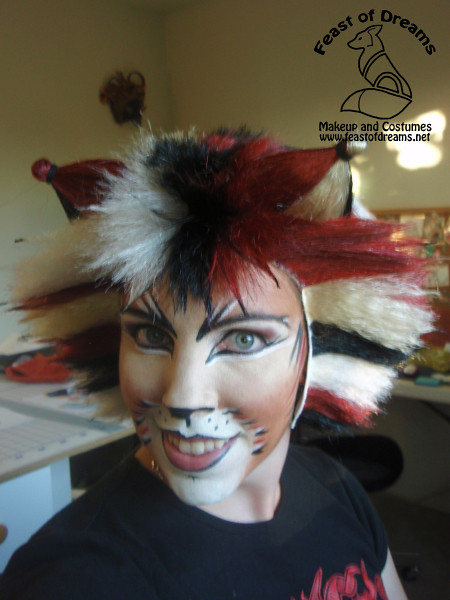In this indoor selfie photograph, a woman is positioned centrally, capturing her face and part of her upper body. She is wearing a black t-shirt and has intricately painted her face to resemble a feline, with a black-painted nose, black-lined lips, and white-painted areas around her mouth. Her face is adorned with tan and brown shades around the cheeks and eyes, mimicking a cat's fur pattern, complete with drawn-on whiskers and dark lines around her eyes. Her head is topped with a hat featuring black, white, and red fur, suggestive of a wig with cat ears. She is smiling and looking directly at the camera. The background reveals a light yellow wall and some indistinct items, possibly indicative of a makeup studio setting. In the upper right corner of the image, a black logo depicting a fox is visible, accompanied by the text "Feast of Dreams" and "Makeup and Costumes" with the website "www.feastofdreams.net".